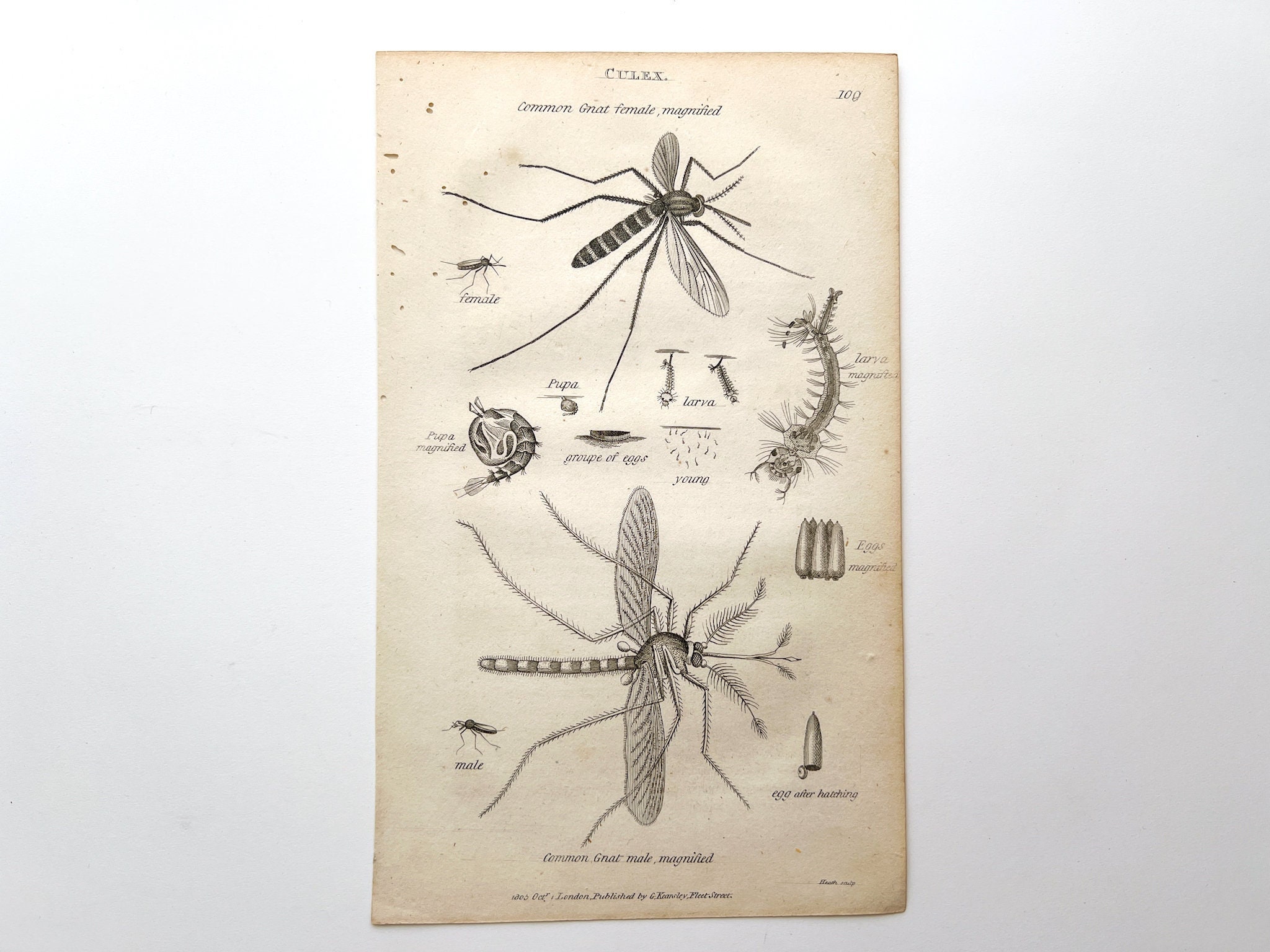This image, taken from an old, slightly faded 1800s biology book, features a detailed infographic of common gnats, specifically a male and female mosquito, each magnified and labeled. The background of the page is an antique, off-white color, giving it an aged appearance. At the top of the page, there is a caption indicating "common gnat female magnified." 

The centerpiece of the image shows large illustrations of both a male and female mosquito, meticulously labeled and showing their distinct physical characteristics, such as long legs and wings. Below these illustrations, the lifecycle of the mosquito is detailed, including diagrams of their pupae, larvae, and eggs, giving clear insight into each stage from young to adulthood. The illustrations are accompanied by somewhat difficult-to-read cursive annotations, typical of old scientific texts. Additional small diagrams highlight specific parts of the insects and emphasize the developmental stages, such as rolled-up pupae resembling tiny balls and squiggly larvae that look like exaggerated eyebrows on a whimsical drawing. On the far right, there are further diagrams, some appearing similar to centipedes due to multiple legs, but all contributing to the comprehensive depiction of the life of a mosquito.